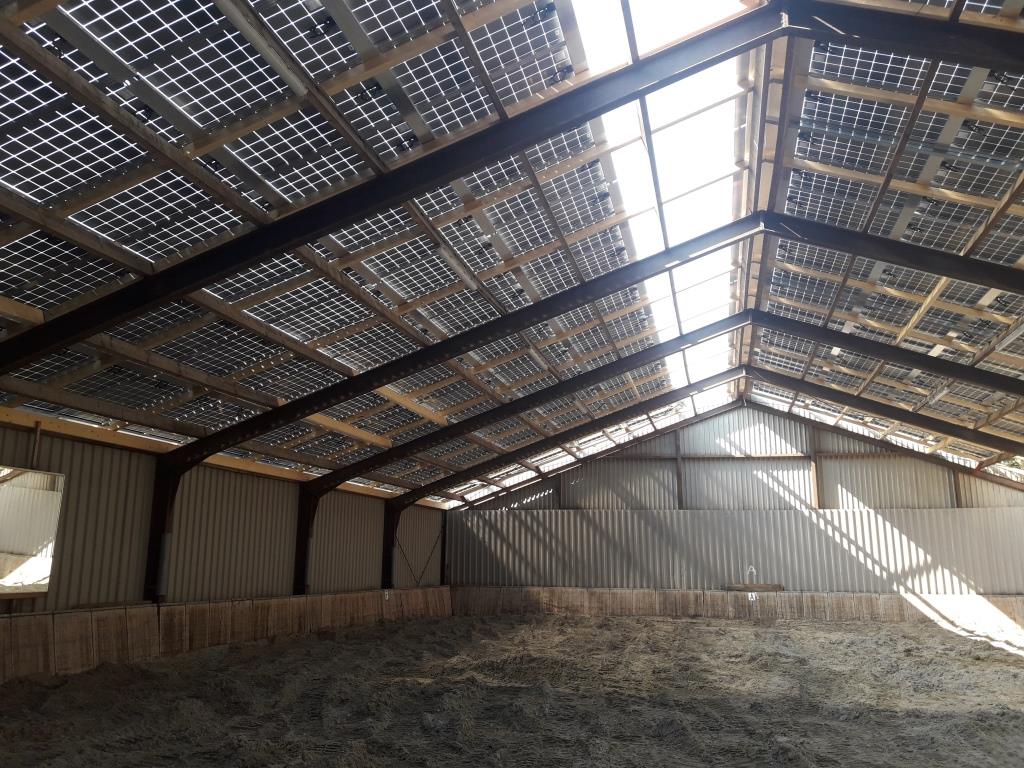The photograph captures the interior of a modern metal barn or greenhouse during the daytime. The structure features a distinctive triangular, sloped roof framed with large black beams and cross beams made of lighter wood. A significant section of the roof is retractable, allowing for sunlight to penetrate and potentially featuring either glass or solar panels. The central part of the roof is currently open, extending from the top to the base, revealing an incomplete ceiling. The walls are composed of light brown corrugated metal, accented at the base with wood panels and cement blocks for protection. The floor is covered in soft, churned-up soil or straw, suggesting a purpose for growing plants or housing animals. The spacious, airy design with retractable elements emphasizes its functionality and adaptability.